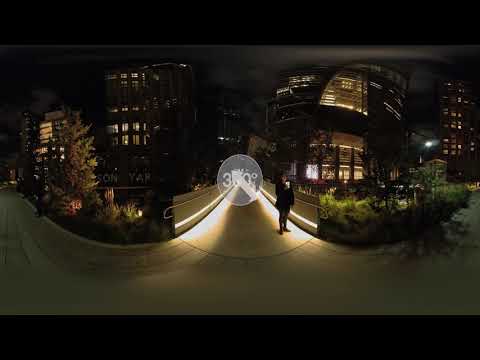In this detailed nighttime scene, a woman stands on a modern, well-lit walkway that resembles a bridge, surrounded by a solid black border. She is positioned near the center, slightly off to the right, engrossed in her phone. The woman has short black hair and wears a black waist-length jacket, Levi blue jeans, and tan boots. The bridge or walkway is flanked by small gardens with lush bushes, trees, and colorful flowers on either side.

Behind the bridge, a cityscape emerges, featuring a mix of residential apartment buildings on the left and larger office buildings with prominent windows on the right. Further in the background, more substantial buildings rise, nearing approximately 20 stories tall. The scenery around the bridge suggests a park-like setting within a residential area, with abundant greenery.

In the center of the image, there's a watermark that reads "360 degrees" in white text within a gray circle, indicating the 3D, 360-degree nature of the image. The overall ambiance is dark, likely indicating it is the middle of the night, accentuated by the artificial lights illuminating the bridge and casting a subtle glow over the scene. The colors visible in the image range from black, gray, and yellow to various shades of green, pink, tan, and brown.